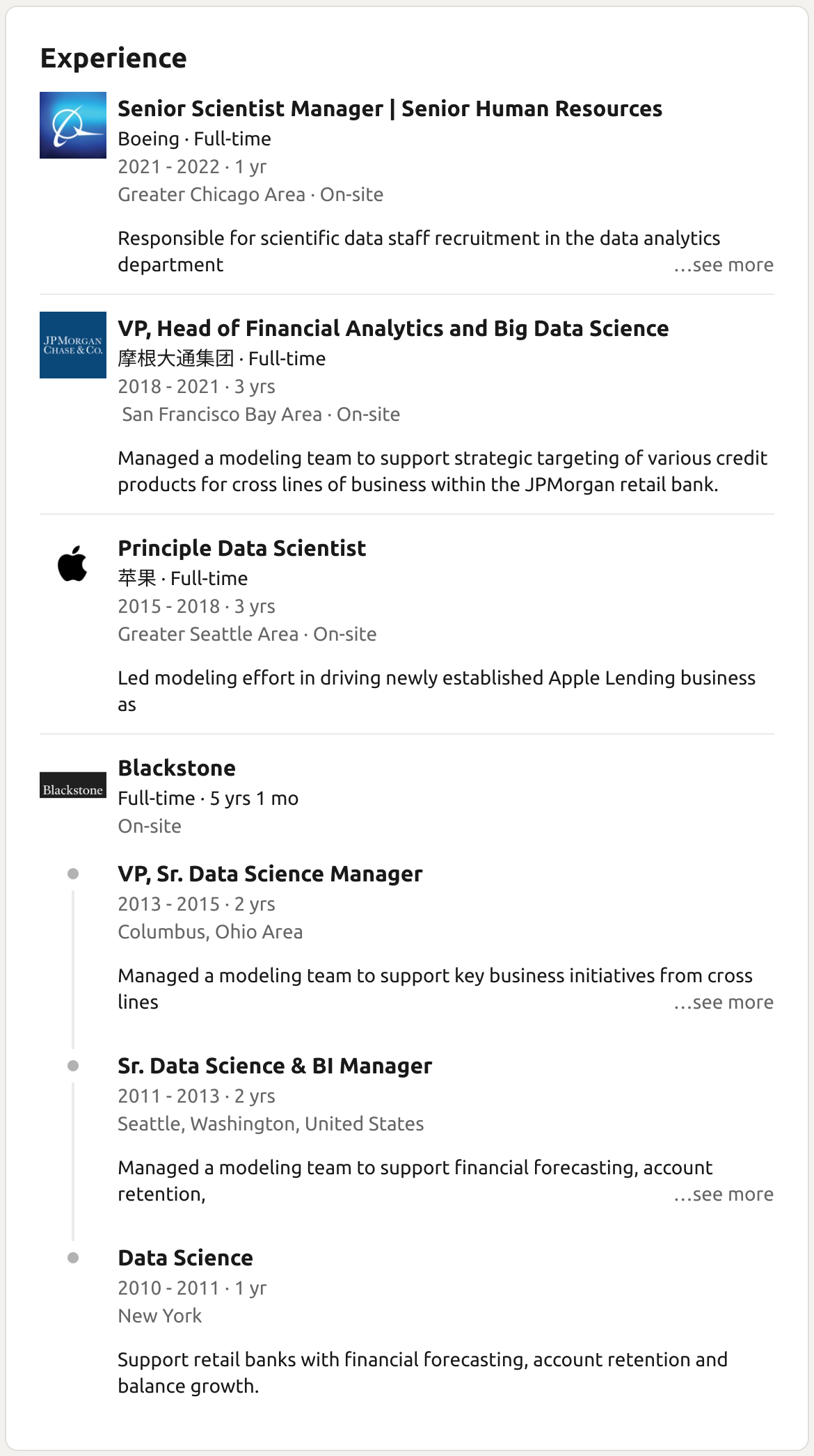Screenshot of a Phone Displaying Professional Resume Details:

At the top of the screenshot, the title "Experience" is prominently displayed in black font. Below this heading, an icon featuring a stylized "Q" with a swoosh around it is visible.

**Role**: Senior Scientist Manager, Senior Human Resources  
**Company**: Boeing  
**Duration**: 2021 - 2022 (1 year)  
**Location**: Greater Chicago Office (On-site)  
**Responsibilities**: Overseeing scientific data recruitment, specifically responsible for the recruitment of staff in the Data Analytics department.

Following this role, there is another section containing the details of a different position:

**Role**: Vice President, Head of Financial Analytics and Big Data Science  
**Company**: (Chinese Name)  
**Duration**: 2018 - 2021 (3 years)  
**Location**: San Francisco Bay Area (On-site)  
**Responsibilities**: Managed and led a modeling team to support strategic targeting of various credit products across different lines of business within JPMorgan Retail Bank.

Additional professional roles are summarized below these entries:

**Role**: Principal Data Scientist  
**Company**: Blackstone  
**Duration**: 5 years

Further entries mention positions such as Vice President, Senior Data Manager at various organizations. The resume details span from 2010 up to the present, showcasing the individual's extensive professional history.

This screenshot captures a comprehensive view of someone's career trajectory, highlighting key roles and responsibilities across multiple prominent companies.